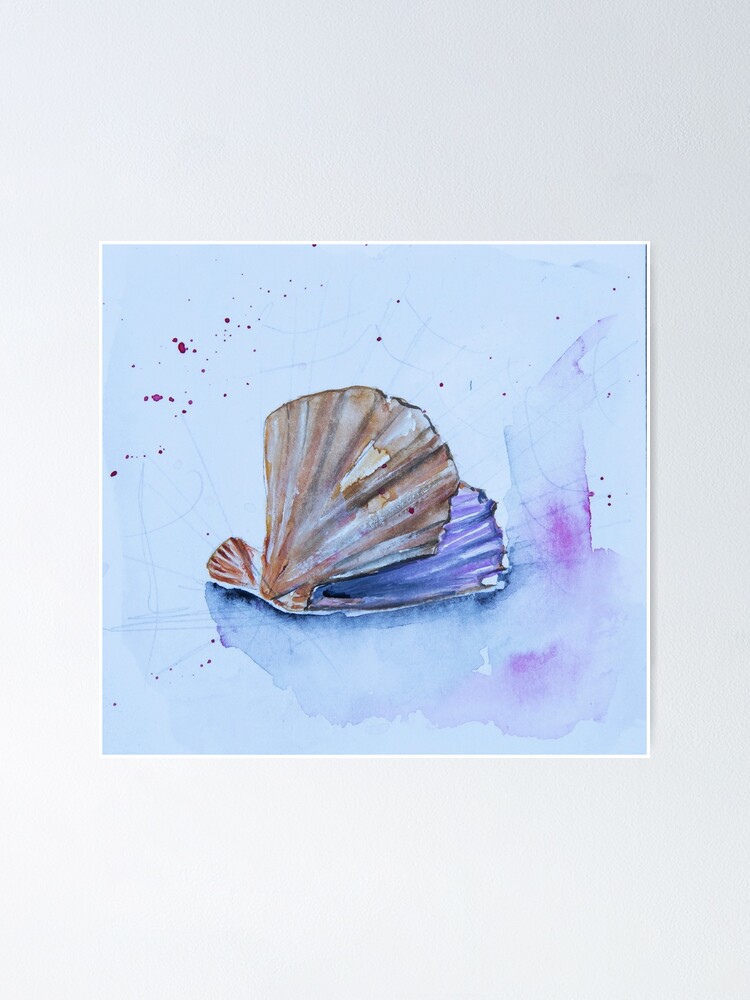This image depicts a detailed watercolor painting of an open seashell displayed on a light blue background. The seashell, fan-shaped and oriented with its open part pointing toward the upper right and the closed part toward the lower left, features an exterior in various shades of brown and tan, transitioning to an intricate purplish hue inside. Red and purple splatters, as well as washes of blue and purple watercolor, accent the blue background, adding a dynamic, textured element to the artwork. The painting, appearing to be on a square canvas without a frame, hangs on a gray off-white wall.